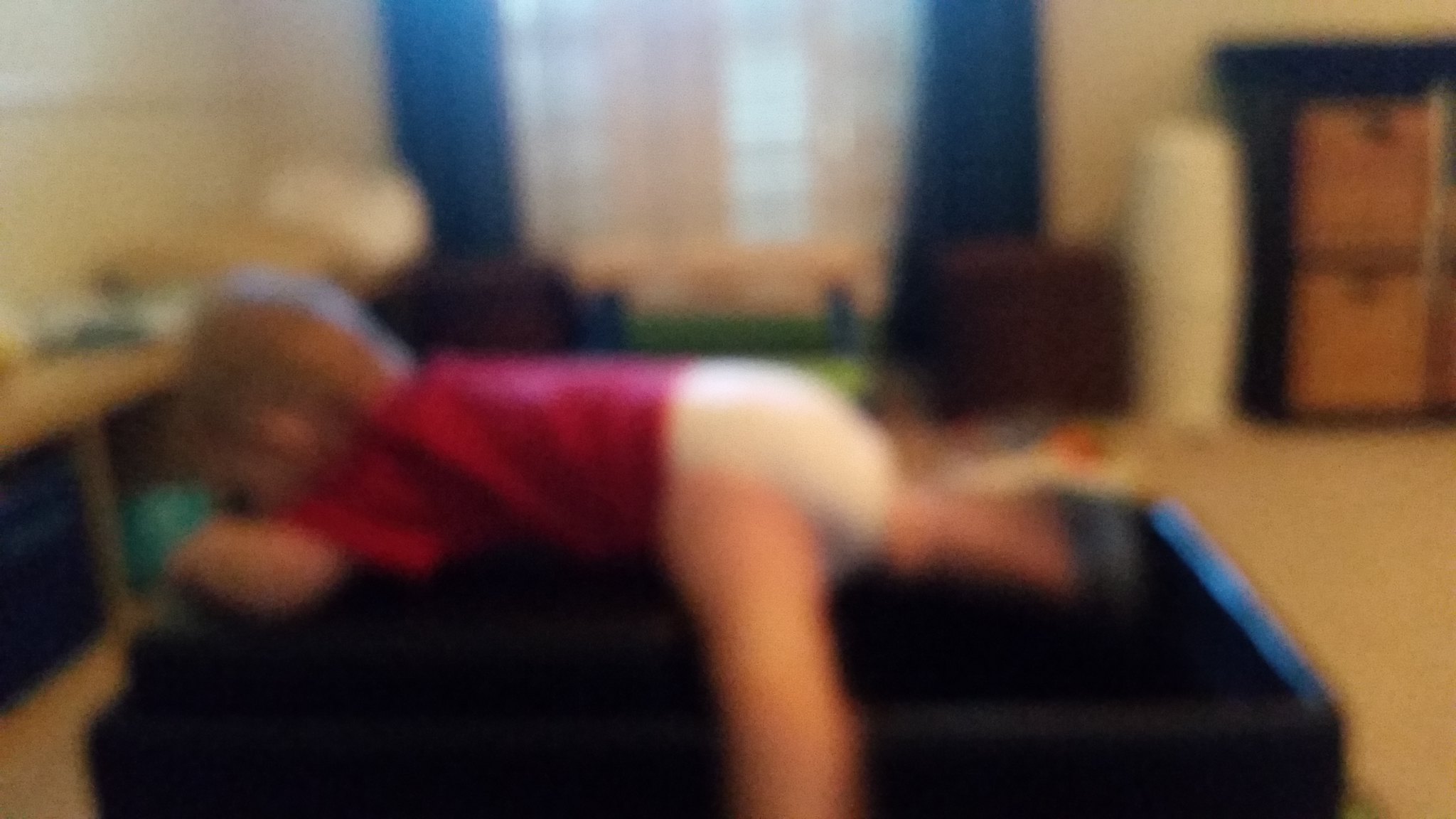In a dimly lit room with beige walls and tan carpeting, a toddler with light brown hair can be seen lying on their stomach on a rectangular blue object with a black border, likely a baby bed or a trampoline. The child, who is approximately around two years old, is dressed in a red or maroon t-shirt and a diaper, with their bare legs indicating they are Caucasian. The room features a variety of furnishings, including a white cylinder fan, brown wicker and wooden furniture, possibly a toy box, and a cabinet with blue items on one side. To the left, a large window is framed by sheer white curtains and thicker blue curtains that are partially open. The overall setting appears to be either a living room or a bedroom, accentuated by additional items like a garbage can, a desk with drawers, and possibly a dresser. The image is notably blurry, making precise details difficult to discern.